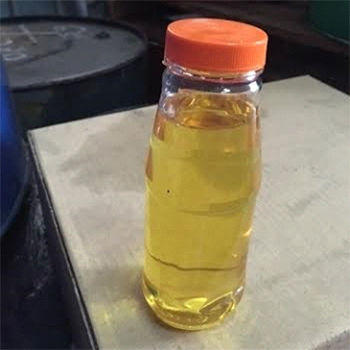The image features a clear bottle with an orange cap, slightly off-centered towards the right and positioned diagonally on a white square surface, likely a countertop or a cushion. The bottle, which is about 80% filled with a yellowish liquid, appears to be upright with its cap on. In the background, to the top left, there is a black barrel or drum, and an edge of a blue barrel is visible on the left. The scene seems to be set in an indoor environment, possibly a warehouse or garage, with a mix of colors including gray, white, black, yellow, orange, brown, and a touch of blue. There is no text or discernible lighting source to indicate the time of day.